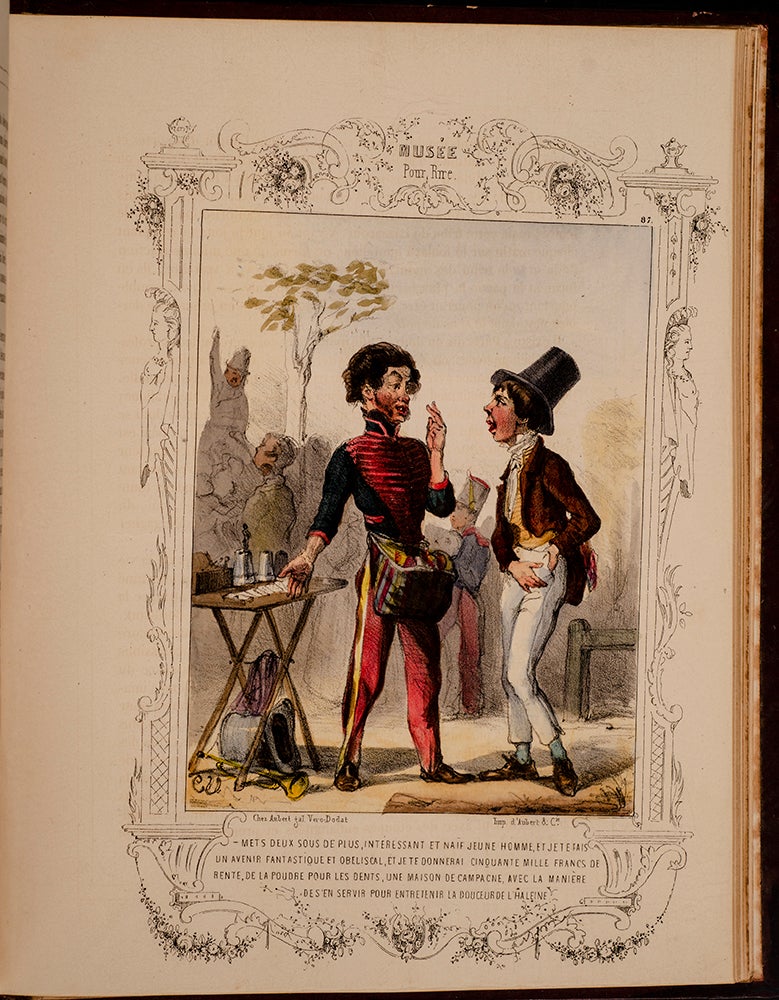This artwork appears to be an antique illustration, possibly from a medieval manuscript, given the yellowed paper and the presence of mold along the edges. The title at the top reads "Musee Pour Rme" in ornate calligraphy, though the meaning of the latter words is unclear. Encased in a dark, ornate border resembling Greek columns entwined with vines, the central image portrays two comical-looking men engaged in conversation. The man on the left, dressed in red pants with a yellow stripe and a red ruffled shirt with black sleeves, stands beside a small folding table adorned with indiscernible items. Facing him is a man with dark hair, wearing a top hat, a maroon jacket, a yellow vest, and white pants. Below the image are four lines of text in French, their contents unreadable, framed by the same intricate design that lines the top and sides of the illustration.